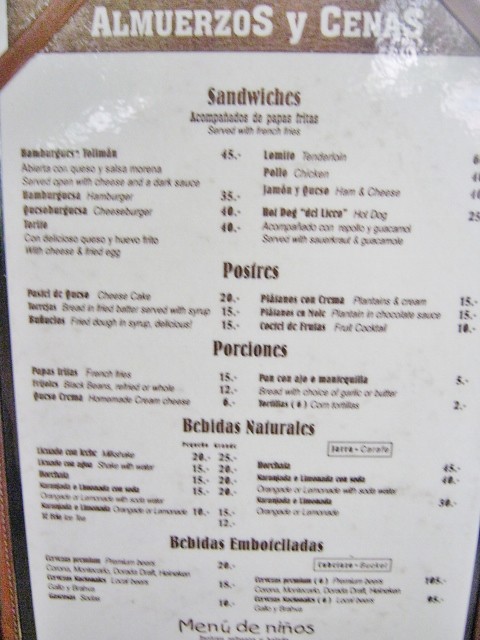The image features a single-page restaurant menu titled "Almuerzos y Cenas," which translates to "Lunches and Dinners" in English. The menu is presented on a white background with dark brown lettering, giving it a clean and elegant appearance. At the very top of the menu, the name of the restaurant "Almuerzos y Cenas" is prominently displayed. The content of the menu is organized into two main columns that list various dishes under clearly defined sections.

The first section on the left side of the menu is labeled "Sandwiches," followed by another section for "Postres" (pastries) and "Porciones" (portions). Due to the blurry and small text, the menu items are somewhat difficult to read, but it is evident that the menu is written in Spanish. Despite the challenges in readability, the menu appears to offer a wide variety of dishes for diners to choose from, showcasing the establishment's diverse culinary offerings.